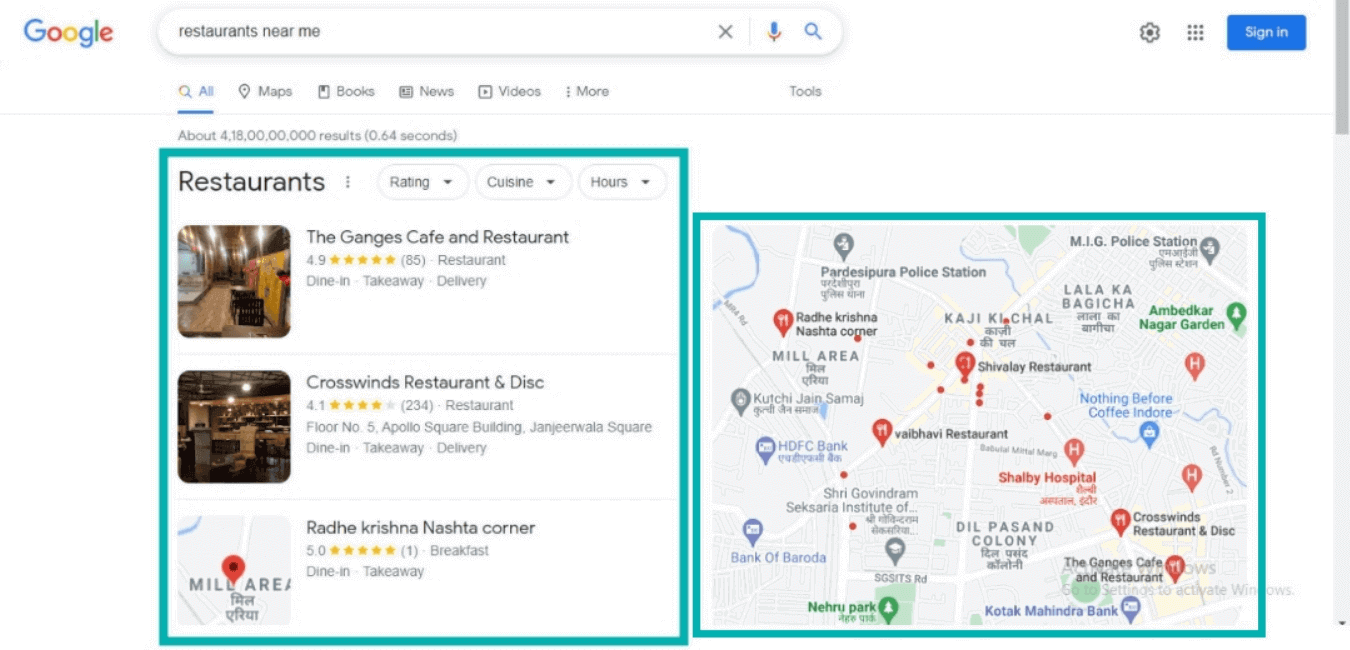This image shows a Google search for "restaurants near me." The search results display a section dedicated to restaurants on the right side and a map on the left side of the screen. Both the restaurant listings and the map are outlined with a prominent blue border. The restaurants listed include "Genji's Cafe and Restaurant," "Crossword Wind and Disk Restaurant," and "Radhi Krishna Nat Tea Corner," all of which appear to be Indian restaurants. The search results suggest that these establishments are located in or near the same area.